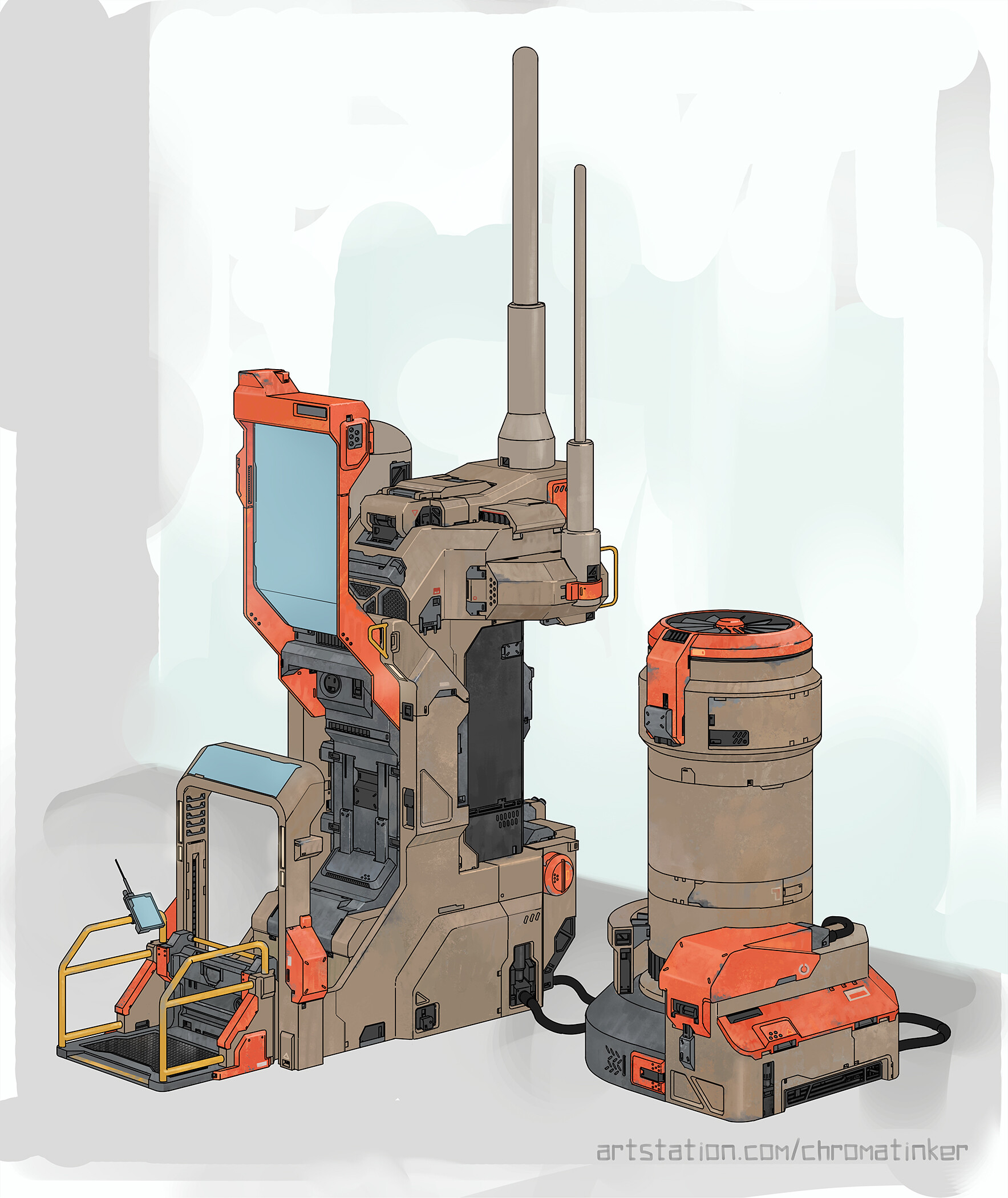The image depicts a detailed digital illustration, seemingly created using computer-aided design. It portrays two pieces of machinery set against a background that combines a light pale mint green wall and a grey floor. The illustration is oriented in portrait mode. The primary machinery, centered in the composition, has a predominantly brown, tan, and orange palette, and features elements that suggest it could be from a futuristic video game. This main machine includes an elevator-like lift for standing, two large antennas on top, and two blue screens outlined in orange. Adjacent to it is a smaller, cylindrical machine with similar brown and orange accents, topped with a large fan. In the bottom right corner, the grey text "artstation.com/Chromatinker" signifies the artist's website.